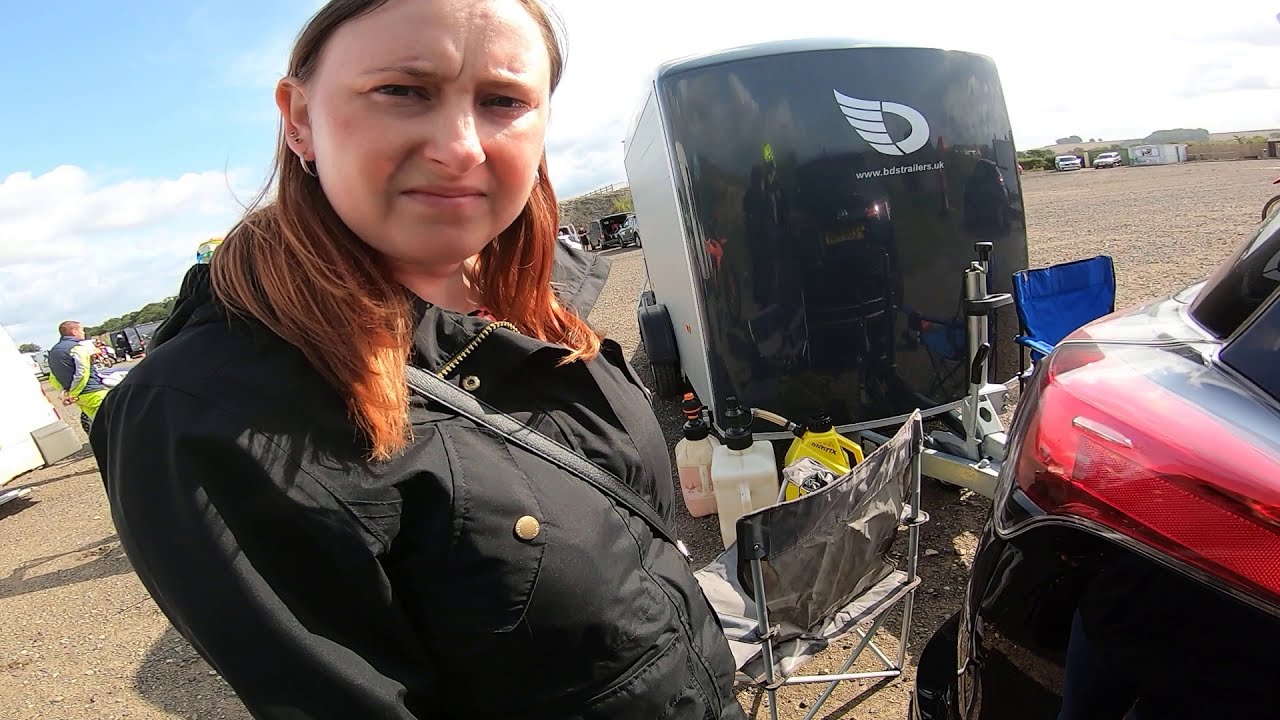A fair-skinned Caucasian woman with red hair combed behind her ears stands and gazes slightly to her left into the camera. Her eyes are brown and somewhat squinted, with closed pink lips and a hint of redness on her cheekbones. She is dressed in a black jacket adorned with gold buttons and a strap running across her shoulder to her waist, likely indicating she has a bag on her other side. Near her right shoulder, there is a shiny black trailer featuring a winged decal and the website address www.beastraiders.uk. 

In front of the trailer, there is an assortment of objects including a yellow bottle with a black cap and a spout, alongside a couple of white-colored bottles. To the right of these items, a fold-out chair is visible on the gravel surface of the parking lot they appear to be in. In the background on the left side, a man dressed in light green pants, a blue vest, and a white shirt stands with his hands behind his back. Further in the distance, there are two parked white cars adjacent to a white building. Additionally, the taillight of a black car is discernible in the bottom right corner near another chair with a blue backrest. The sky is mostly cloudy with a small patch of blue in the top left corner, shining sunlight emphasizing a glare across the scene.